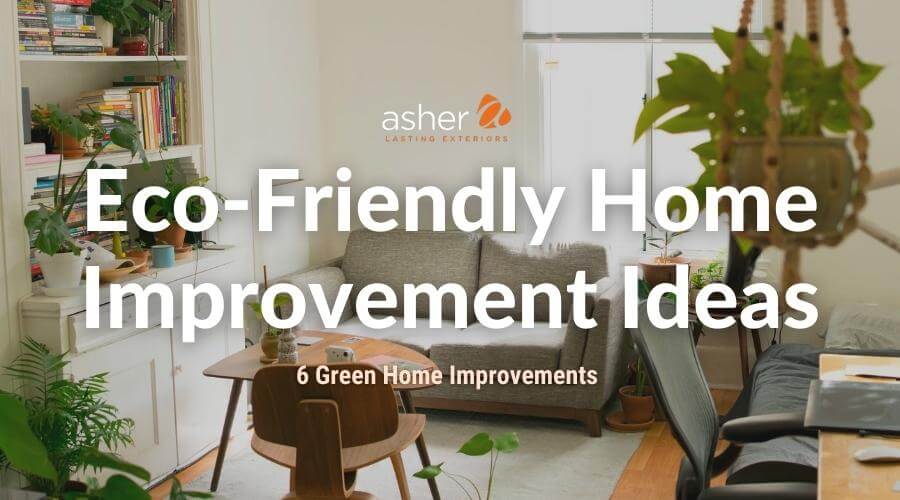The image is a detailed rectangular banner designed for an online blog or listing. It features a color photograph of a cozy, eco-friendly home office or studio room, emphasizing sustainable living. The banner, oriented in landscape, showcases a combination of modern interior design elements and text overlays in various shades of white, peach, and orange.

Dominating the center of the banner, bold white text reads "Asher Casting Exteriors," followed by "Eco-Friendly Home Improvement Ideas," and a smaller, peach-colored line stating "Six Green Home Improvements." The "Asher" logo stands out at the top center, accompanied by an orange, broken-up triangle beside the letter 'A'.

The background photograph captures a room with a harmonious blend of comfort and functionality. On the right side, there is a light brown wooden desk with a closed laptop, paired with a black office chair. In the upper right corner, a hanging plant in a beige macrame holder adds a touch of greenery. Below, a low bed with a black sheet and a pillow is visible next to the desk. 

On the left side, the room features a white-walled built-in bookshelf filled with books and plants. Below the bookshelf, at the bottom left, stands a vibrant green potted fern. Just in front of the bookshelf, a gray loveseat sits on a light gray rug, completing the cozy ambiance of the room. The overall style of the banner blends photographic realism with impactful textual elements to create an inviting and informative visual.